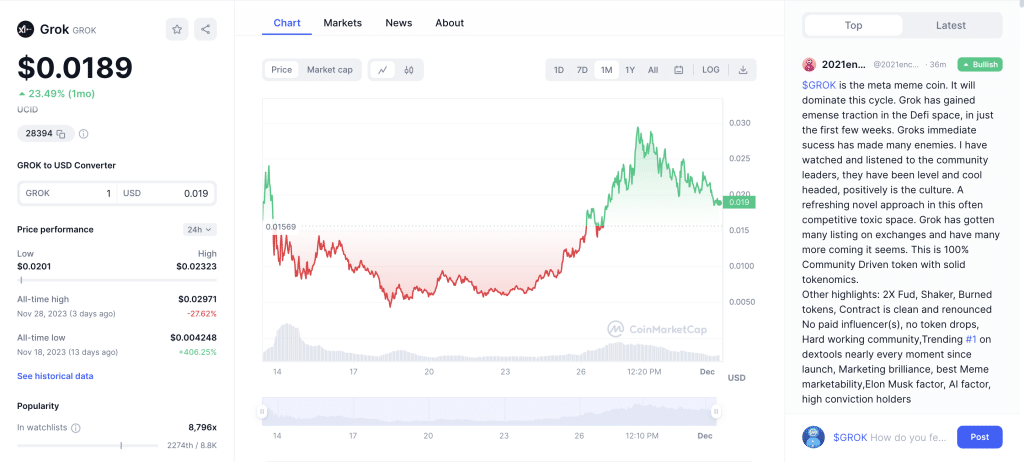This image is a detailed screenshot of a cryptocurrency charting website for a digital currency called Grok. In the top left corner, the name "Grok" is prominently displayed. Directly below the name, the current price of Grok is shown as $0.0189, along with a significant monthly increase of 23.49%.

Beneath the price and percentage increase, there is an array of additional data. This includes a calculator designed to convert Grok into US Dollars, the 24-hour high and low prices, as well as the all-time high and low values for the cryptocurrency. The website also displays information regarding the popularity of Grok.

Dominating the center of the screen is a detailed price history chart for Grok spanning one month, providing a visual representation of its price fluctuations.

On the right side of the screen, there is a section dedicated to user posts and comments about Grok. A recent post by a user is highlighted, providing a description of what Grok is and further discussing its attributes.